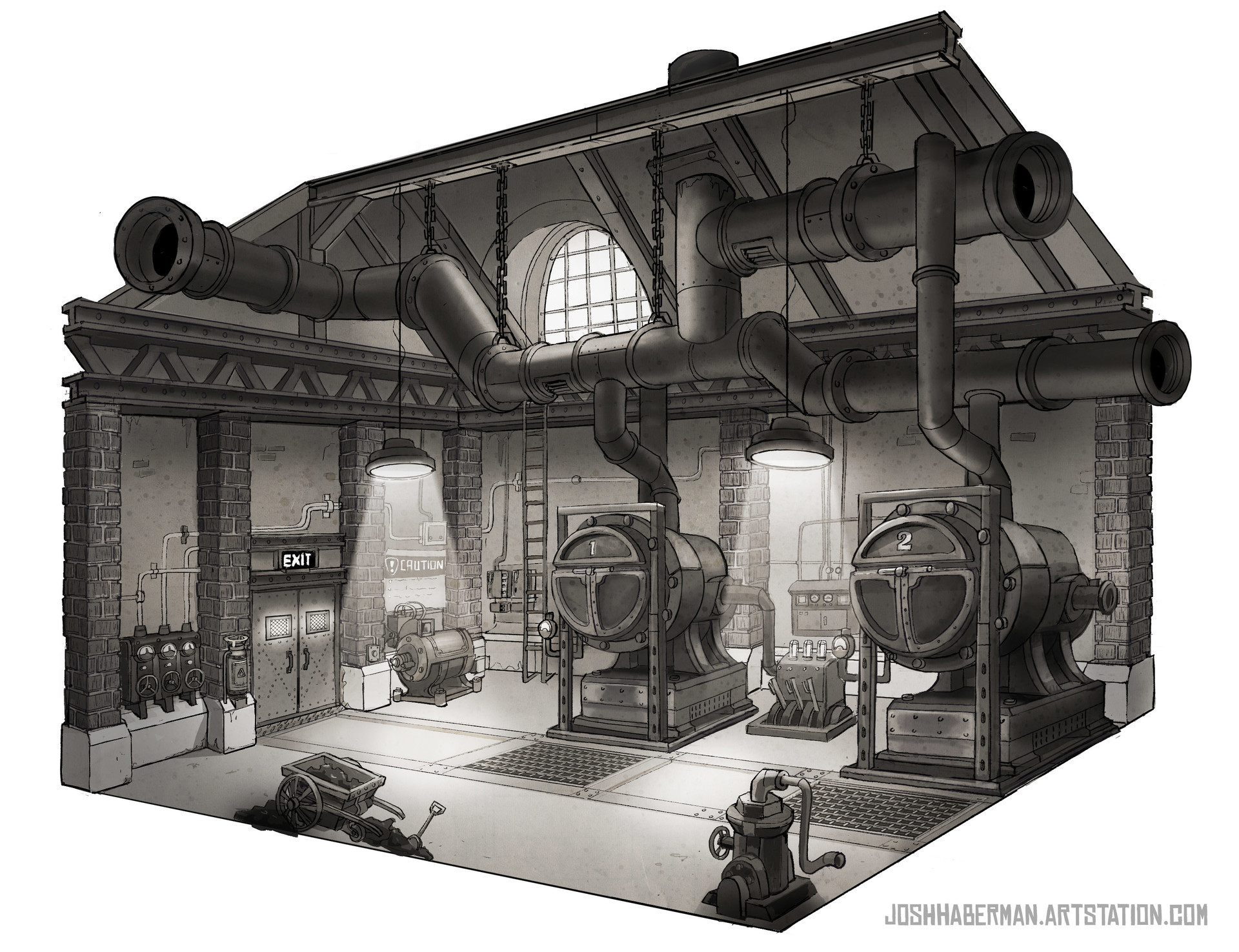The black and white drawing, reminiscent of a comic book or graphic illustration, depicts the intricate interior of a mechanical factory with a strong sense of depth and perspective, viewed from the bottom right corner. The ceiling is a tangle of large pipes stretching left to right, with chains and two bright pendant lights illuminating the scene. Dominating the room are two large, numbered machines, labeled "1" and "2," connected to substantial vents leading through the ceiling. Between the vats lies a control device with various levers and gauges.

On the left side of the room, a set of double doors marked with an "Exit" sign is positioned beneath a caution sign, providing a focal point for escape. The floor features built-in openings and on the far left, a ladder leads up to an upper level. The walls are characterized by brick pillars and brick fascia, adding a rustic texture to the industrial setting. Additional details include a wooden barrel, a shovel, and what appears to be a pump, contributing to the factory’s busy and operational ambiance. The bottom right corner of the image is watermarked with "joshhaberman.artstation.com," crediting the artist and their portfolio.